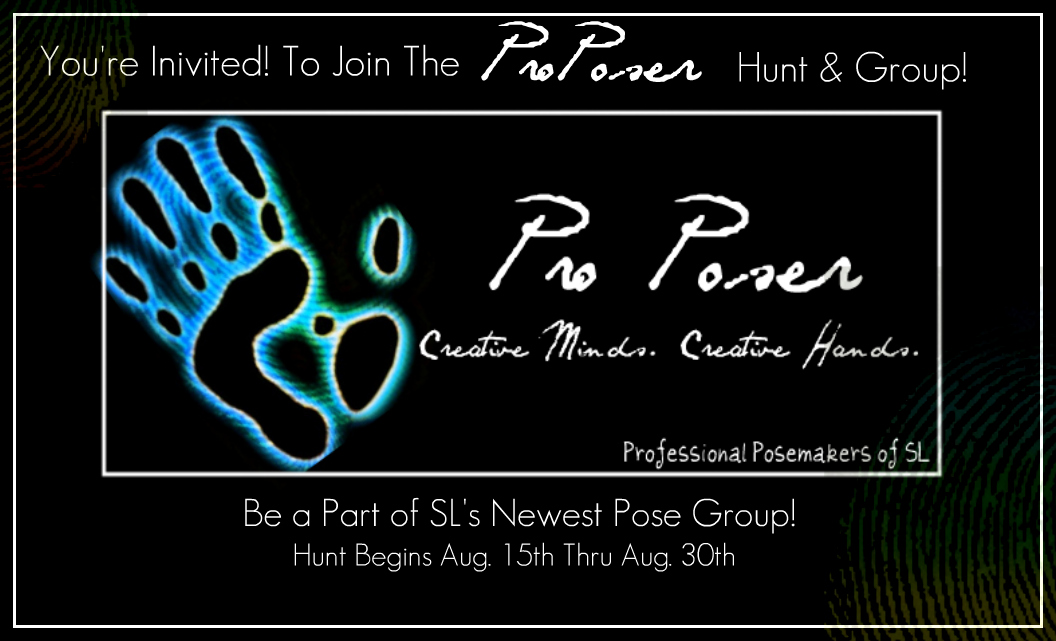The image features an advertisement with a black background, accented by a thin white border that frames the entire composition. At the top of the image, white text reads, "You're invited to join the Pro Poser Hunt and Group." Centered in the middle is a prominent rectangular box, also outlined in white. 

On the left side within this box, there is a striking handprint rendering, resembling a thermal image with black fingers and shades of blue and green surrounding the palm and thumb, as if pressed against a glass pane. To the right of this handprint, in white text, are the words, "Pro Poser," followed by a tagline: "Creative Minds, Creative Hands, Professional Pose Makers of SL."

Beneath this central rectangle, in the middle, additional white text invites viewers with, "Be a part of SL's newest pose group." Directly below that, it announces the event dates: "Hunt begins August 15th through August 30th."